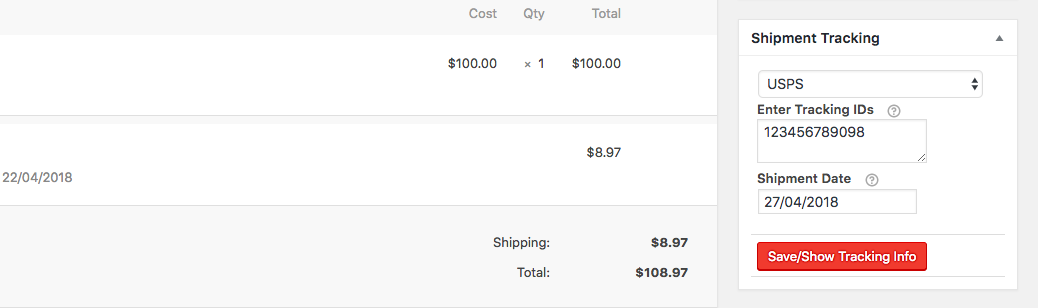The image depicts an online checkout page from a shopping website. The interface is designed with a clean white background, accented by light gray elements for a subtle contrast. 

At the top of the page, there is a summary of the purchase:
- **Cost**: $100
- **Quantity**: 1
- **Total**: $100

Below this, there is additional information:
- **Date**: 22/04/2018
- **Balance**: $8.97
- **Shipping**: $8.97
- **Grand Total**: $108.97

To the right of the purchase summary, there is a section for shipping and tracking information, which includes:
- **Shipping Method**: USPS
- **Tracking ID**: 123456789098
- **Shipment Date**: 27.04.2018

Below the tracking information, there is a prominent red button labeled "Save / Show Tracking Info".

The photograph is slightly cut off, limiting the full context, but it clearly shows an individual finalizing an online purchase for an item priced at $100 with an additional shipping cost of $8.97.